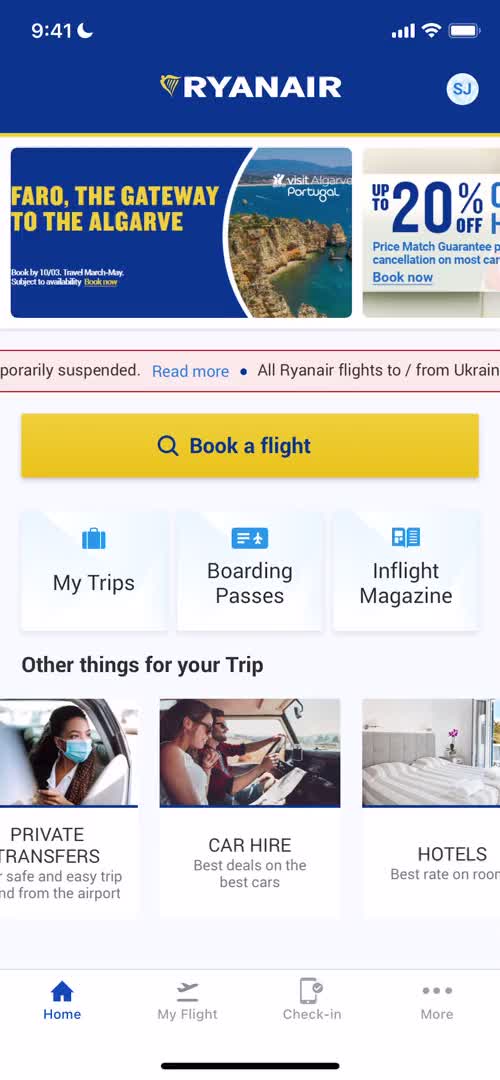The image is a screenshot from a cell phone displaying the Ryanair mobile app. At the top of the screen, the Ryanair brand name is prominently featured in uppercase letters. Below the header, there is a promotional banner for "Fargo: The Gateway to the Algarve" advertising up to 20% off, although a red bar with "Temporarily Suspended - Read More" indicates that flights to and from Ukraine are currently halted.

Further down the screen, a prominent button labeled "Book a Flight" is visible for users wishing to make travel arrangements. Underneath, three distinct sections labeled "My Trips," "Boarding Passes," and "In-Flight Magazine" are presented in square icons.

An additional area titled "Other Things for Your Trip" offers options for "Private Transfers," "Car Hire," and "Hotels," each accompanied by respective images: a woman wearing a blue mask in a vehicle for "Private Transfers," a couple driving for "Car Hire," and a hotel room bed for "Hotels." The bottom part of the screen includes several more icons, though their specific details are not provided in the caption.